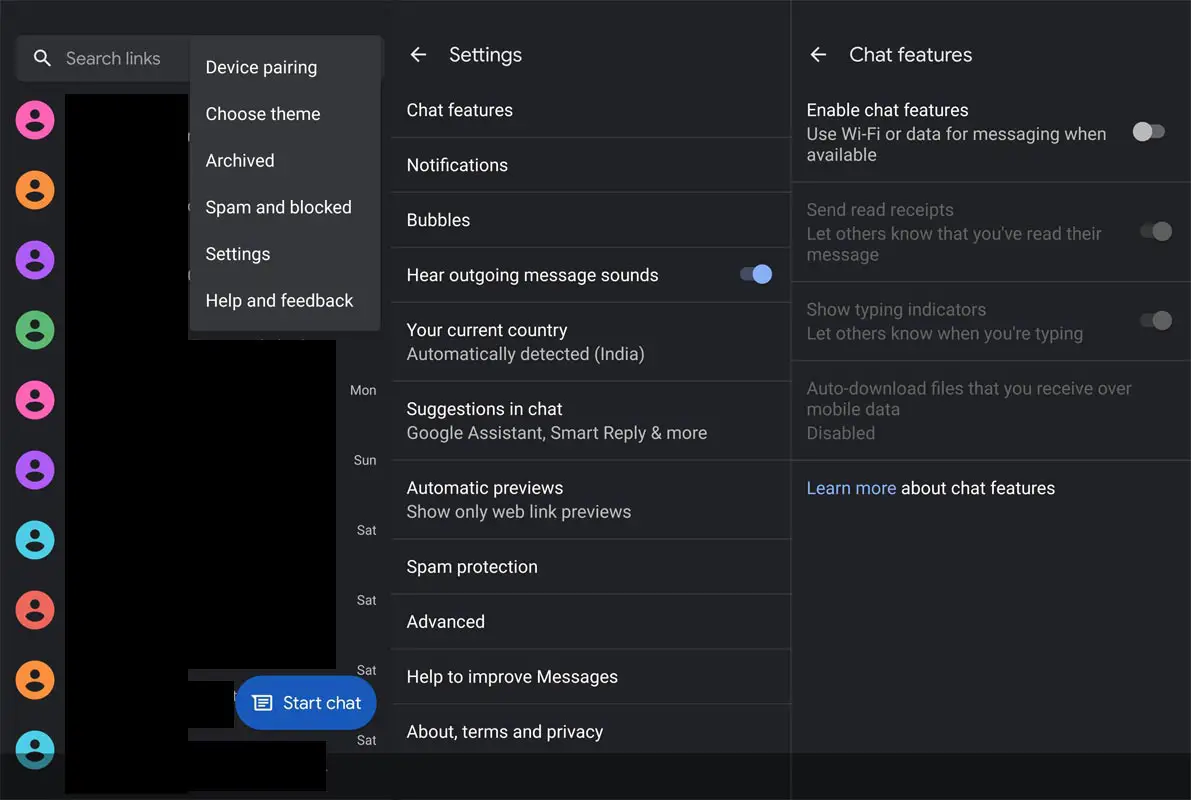The image showcases a comprehensive array of messaging app settings and features. On the left side, there's a search bar accompanied by a vertical list of various profile-like icons stretching to the bottom of the screen. 

At the top center, the interface includes options for device pairing, theme selection, archiving, spam and blocking features, access to settings, and help and feedback. Near the bottom center, there's a conspicuous "Start Chat" button. Adjacent to this, there are options and toggles for settings such as chat features, notifications, and bubbles.

In the central portion of the image, several toggles and links for different settings are shown: 
- Outgoing messages configured to the right
- Automatic country detection, set to India
- Chat suggestions, including Google Assistant and smart replies, and various other settings are listed such as 
   - Automatic previews (show only web link previews)
   - Spam protection
   - Advanced settings
   - Terms of privacy

To the right, there's an arrow pointing to a section labeled "Chat Features." This section includes various settings such as:
- Enabling chat features to use Wi-Fi or data for messaging when available
- Send read receipts
- Show typing indicators
- Option for auto download of files received over mobile data, which is currently disabled
- A link to learn more about chat features

The entire interface is set against a gray background, providing a clean and organized look.